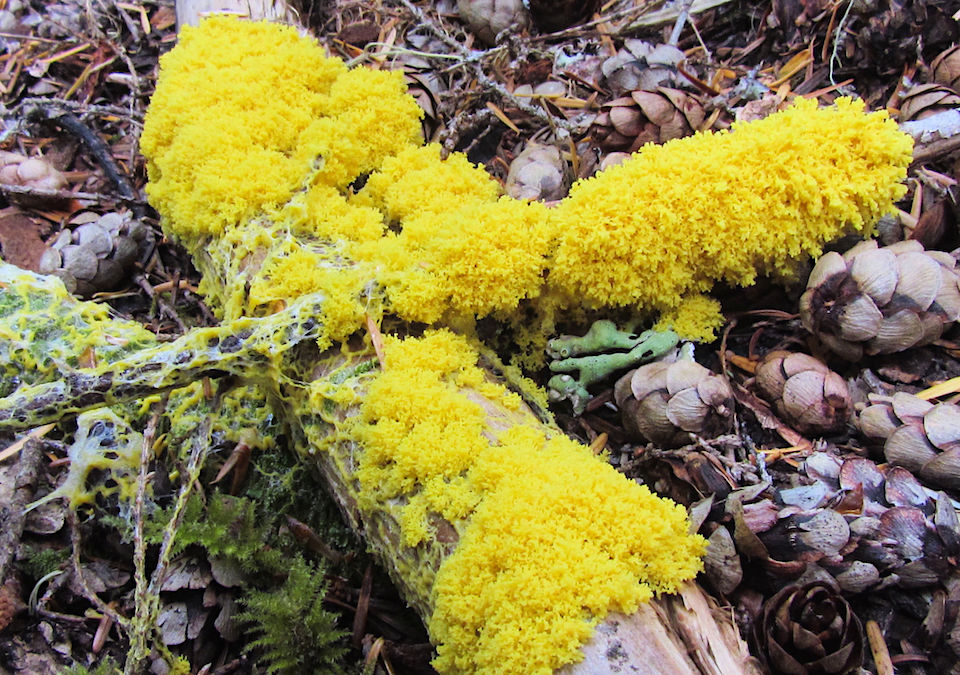This professional photograph, taken in the wild, showcases a richly detailed forest floor scene. Dominating the composition is a decaying tree stump and several wooden branches interspersed with dense yellow fungus or moss, which appears bright and sponge-like, almost resembling finely grated cheese. The vivid yellow growth is contrasted strikingly by muted earth tones and a mix of organic matter, including pinecones with unusually small scales, green ferns, dead branches, and rich soil. Some of the wood features additional white fungi, resembling delicate spider webs. The arrangement includes a larger limb running from the top left to the bottom middle, intersected by a thinner branch, both heavily adorned with the bright yellow fungi, exuding a sense of life overtaking decay in a serene, natural environment.